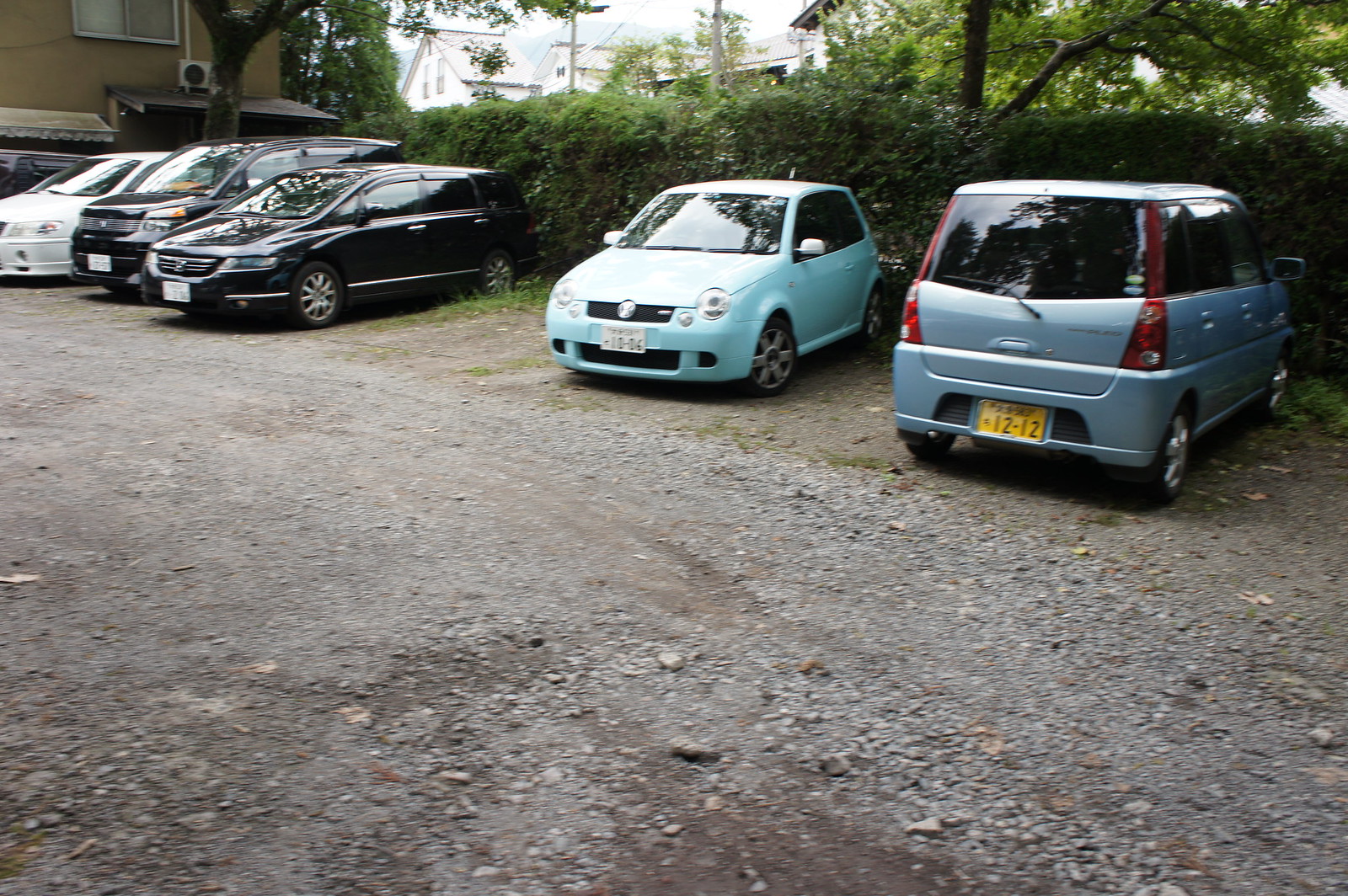The photograph depicts a gravel parking lot with a mix of packed stones and loose gravel, likely situated next to a residence or apartment complex. Positioned in a row, five compact vehicles are parked along what appears to be the right side of the lot, backed up against a tall green hedge. The vehicles, mostly small and boxy, include a light blue minivan, a very pale blue compact car, two black vehicles—possibly an SUV and a minivan—and a white car. One of the black vehicles is notably parked facing outwards while the rest face the hedge. The background features tall trees jutting out from the hedge and several houses with steep roofs, enhancing the daytime setting. On the left side, there stands a tan-colored house or residence with an adjacent tree. The license plates suggest a location that could be in Japan or China.